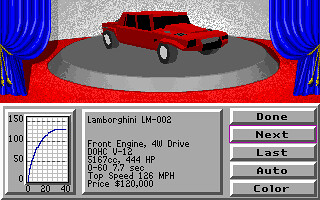This image captures a nostalgic screenshot from an old video game or computer software, characterized by its blocky, low-resolution graphics. Dominating the upper half of the screen is a vibrant red Lamborghini LM-002, impressively displayed on a raised grey circular platform. The platform itself rests on a luxurious red carpet, adding an elegant touch to the presentation. Flanking the car on both sides are grand, deep blue curtains, creating a dramatic, stage-like effect.

The lower portion of the screen is divided into three distinct sections. The leftmost section features a detailed graph, though the specifics are not clear at this resolution. The middle section contains vital information about the Lamborghini LM-002, including its price, speed, and horsepower. The third section along the bottom is a row of interactive buttons labeled "Done," "Next," "Last," "Auto," and "Colour," presumably for navigation and customization within the game or software.